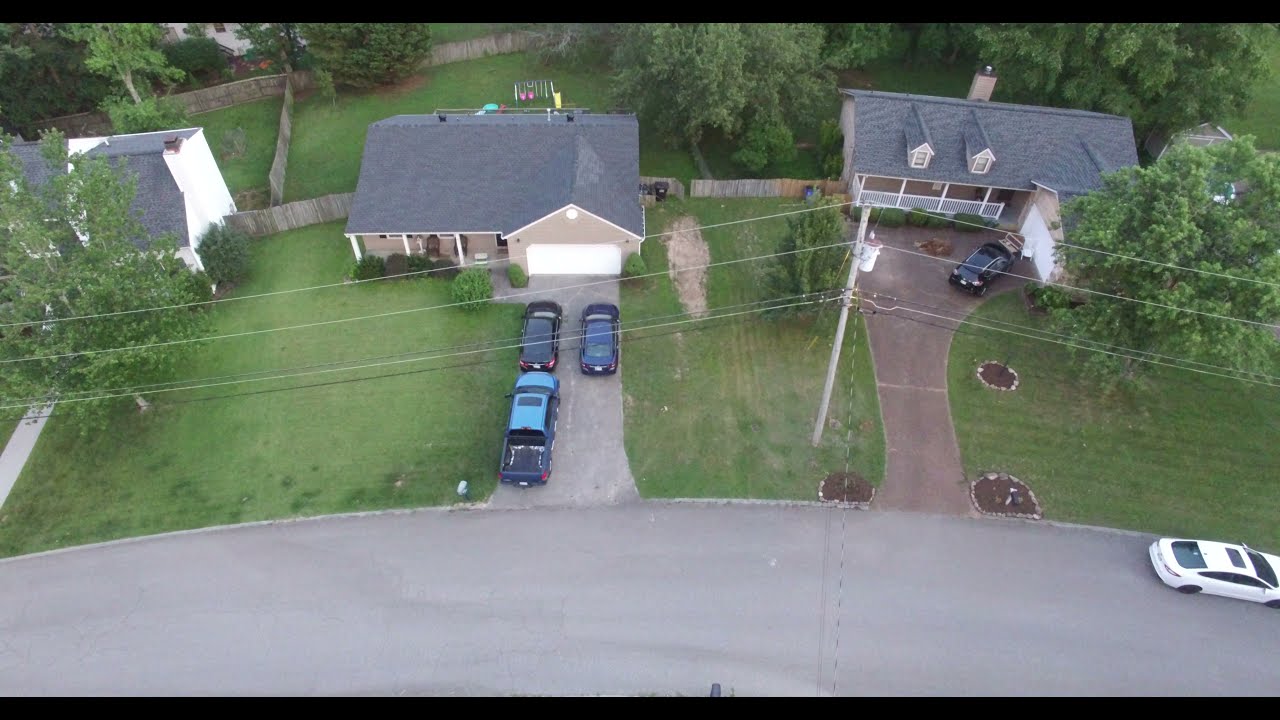The aerial color photograph depicts a suburban neighborhood with three distinct homes, captured in landscape orientation. Each house is surrounded by lush green trees and enclosed by fences in the backyard. The central residence, a single-story structure with brown paint and a gray roof, features a white garage and a driveway where a truck and two cars are parked. This home also has a backyard swing set. To its left, partially obscured by a tree, is another single-story home with a gray roof and a white exterior. On the right, the third house also has a single story with a brown exterior and white garage, and a car parked in the driveway and a white car at the curb.

A gray curved street section runs along the bottom of the image, connecting the residences. Power lines are visible in the middle of the scene. Large trees provide shade and greenery both in the front and backyards of these homes, contributing to the lush suburban atmosphere. The detailed and realistic style of the photograph creates a vivid representation of this residential community.